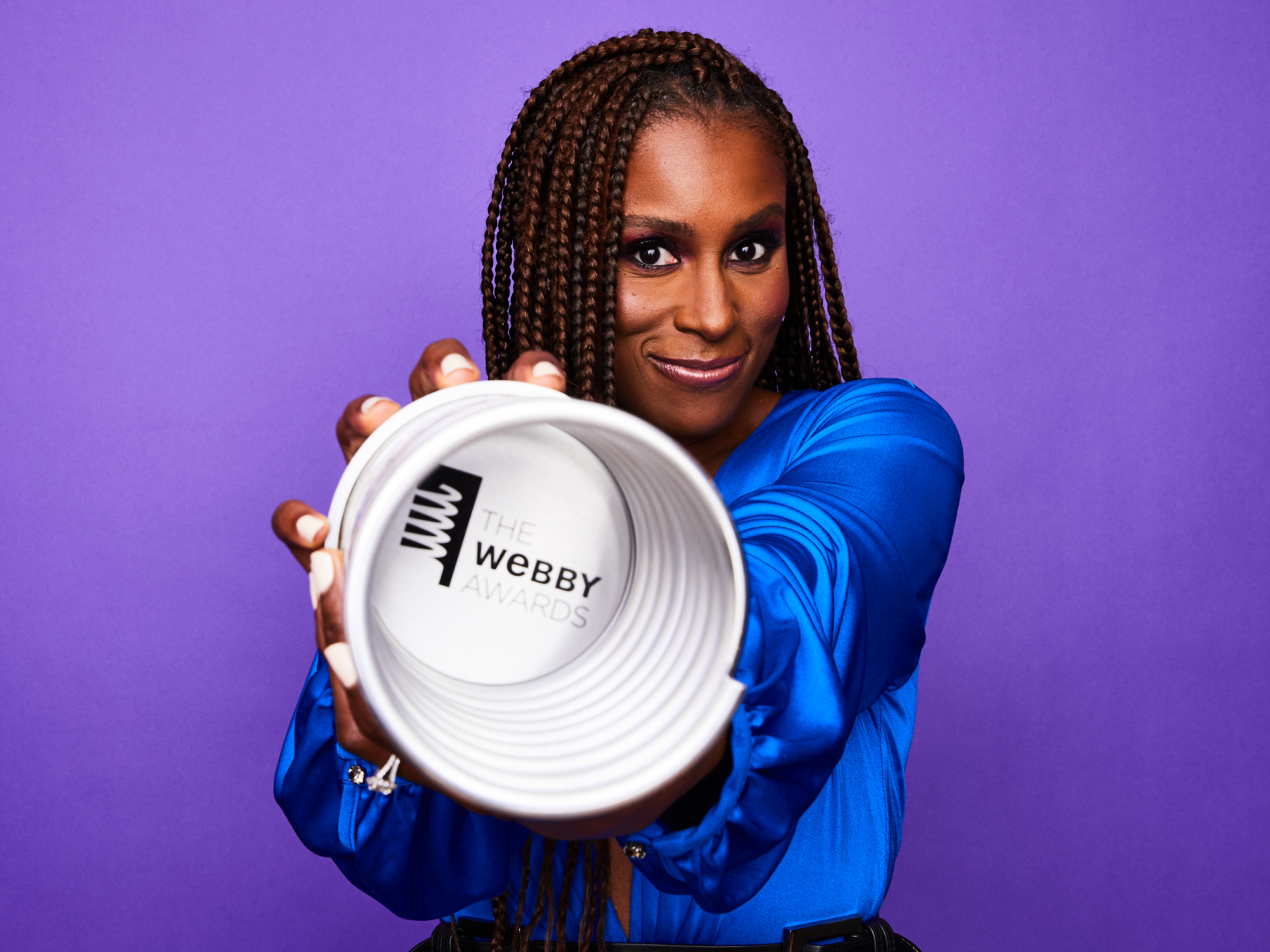The photograph features Issa Rae, celebrated actress and advocate for African American representation in media, best known for her work on "Awkward" and "The Misadventures of Awkward Black Girl." She is pictured holding a white, cylindrical cup with both hands, prominently displaying the inscription "The Webby Awards" at its base in black text. Her dark brown skin contrasts elegantly with her outfit, which consists of a dark blue silk blouse with cinched wrists and dark-colored pants. Issa's black hair is styled in braids, and she is smiling while looking directly at the camera. The background is a striking purple gradient, lighter in the top left corner and transitioning to a darker shade towards the bottom right, likely due to the photograph's lighting and shadows.